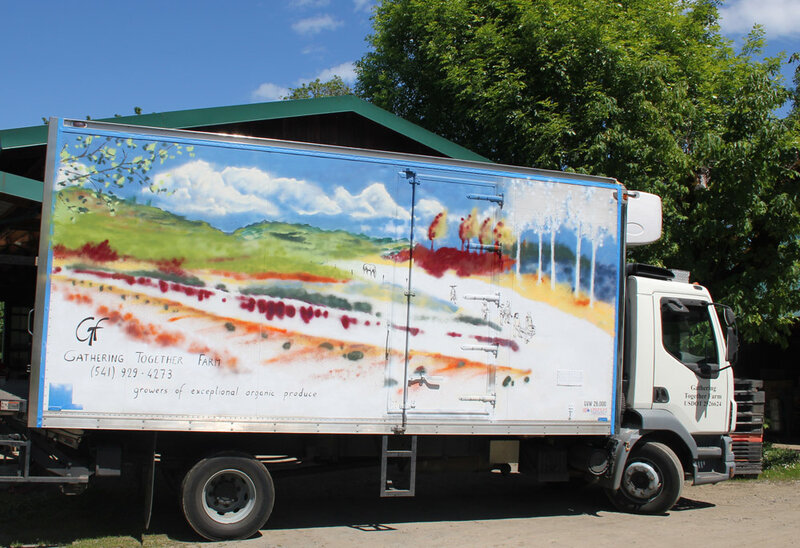The photograph captures a large white box truck parked in front of a house featuring a triangular green roof. The road it sits on is a gray-black asphalt, and a deciduous tree with abundant green leaves stands prominently to the right side of the house. The truck’s front tires are turned, suggesting a maneuver. The side of the truck showcases a minimalist painting depicting a countryside landscape with vibrant colors such as red, yellow, blue, white, green, and orange. The scene includes a blue sky with scattered clouds, green rolling hills, white and red trees, and rows of crops resembling an orchard. On the right side of the illustration, there are farmers walking along a road. The lower left part of the artwork features the letters "G" and "F", along with the text "Gathering Together Farm" and the phone number 541-929-4273. Below this, the words "Growers of Exceptional Organic Produce" are prominently displayed. Just behind and to the right of the truck, some gray plastic boxes are stacked. The detailed depiction on the truck and the surrounding setting creates a picturesque and vibrant scene that suggests the agricultural theme of the farm.